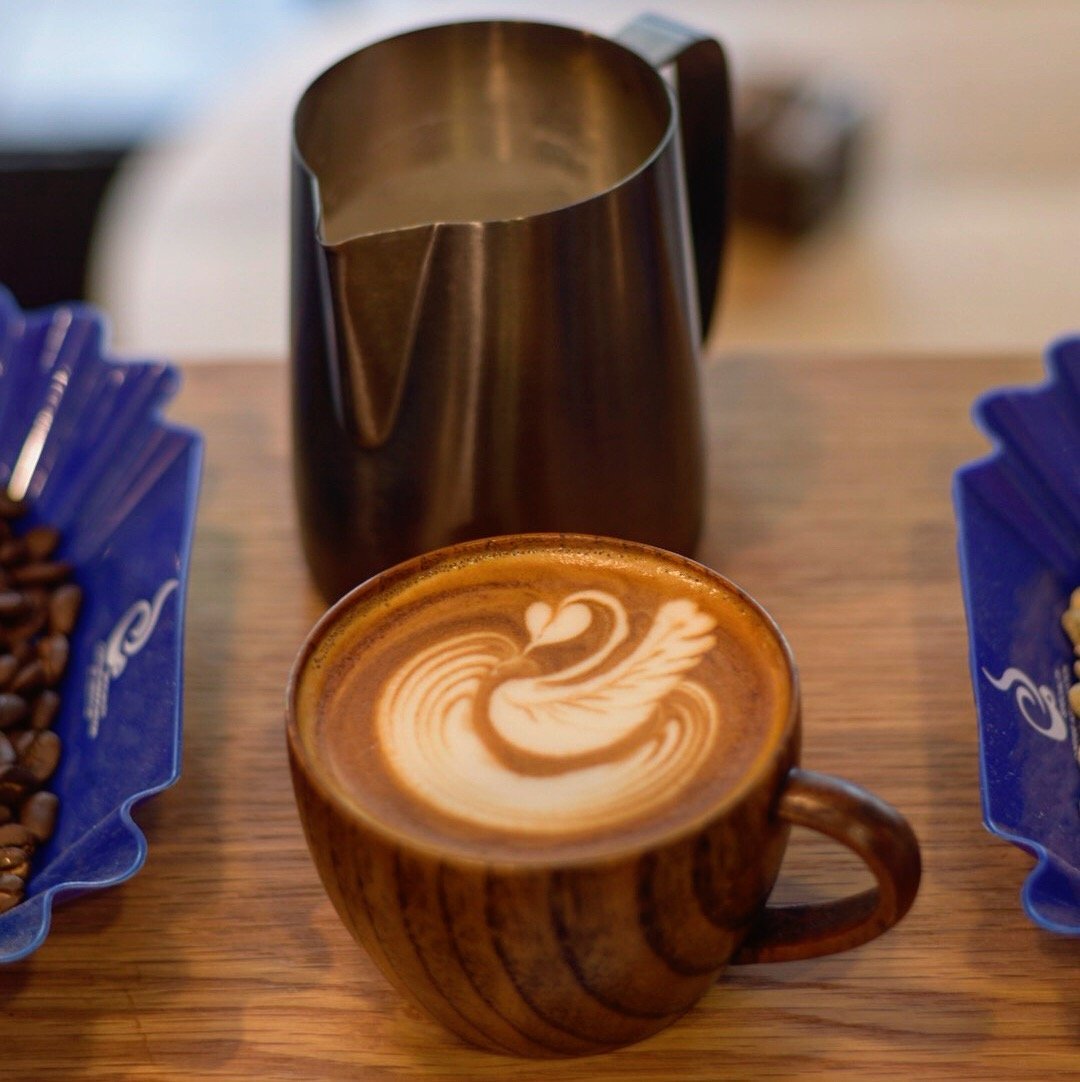This image showcases a meticulously arranged coffee display, likely set in a café. The centerpiece is a short mug of cappuccino featuring intricate latte art resembling a swan with visible feathers and a heart. The cup is positioned centrally at the lower middle of the frame, with the handle to the right. Flanking the coffee mug are two blue trays with raised sides, both containing coffee beans. Directly above the coffee cup is a larger creamer jug, possibly twice the size of the mug, used for pouring milk. All of the items rest on a rich brown wooden table. The color palette includes shades of silver, blue, brown, and white, creating a harmonious and inviting atmosphere. The blurred background suggests the setting is near a window or possibly outdoors, adding to the café ambiance.